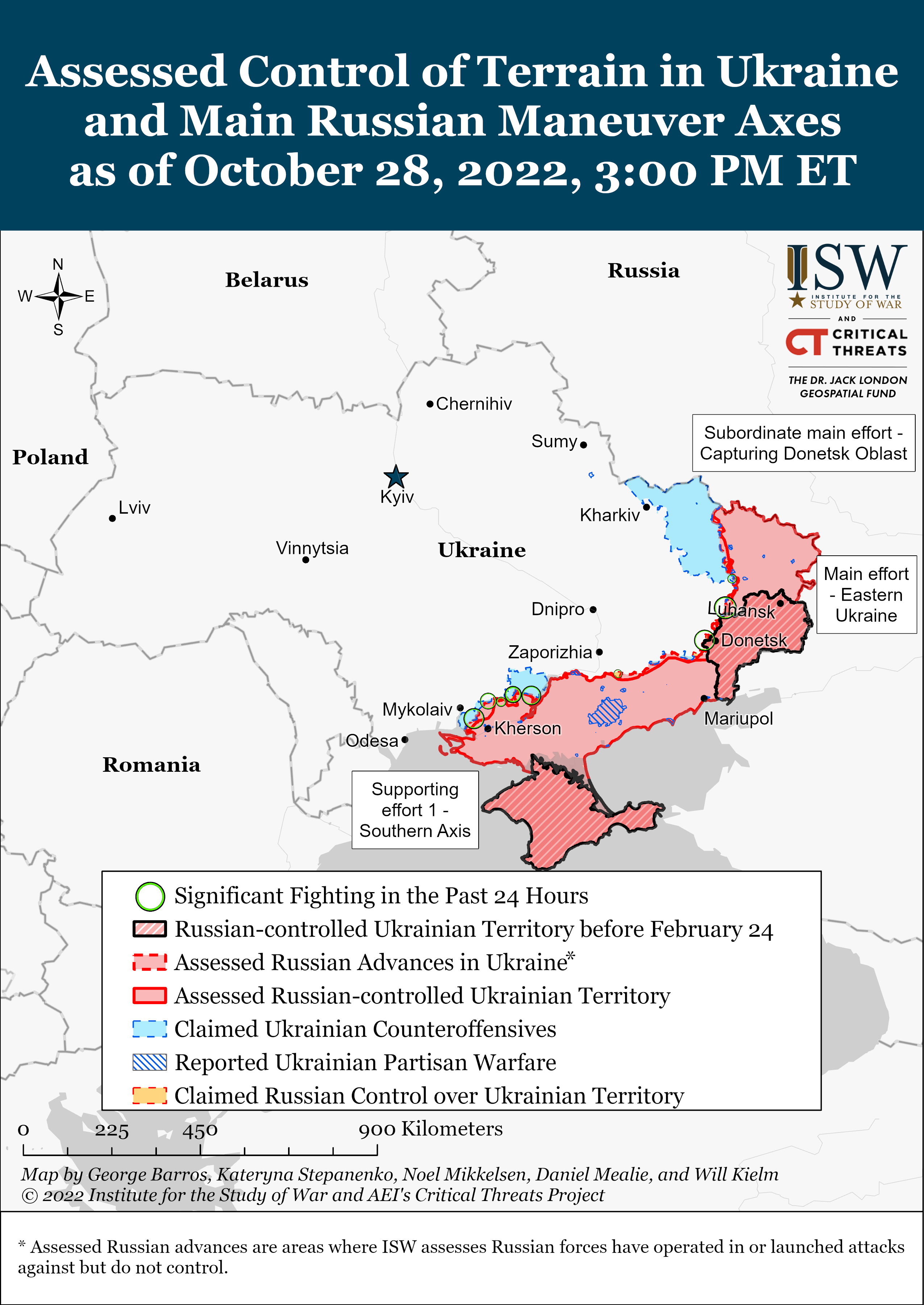The image is a detailed map titled "Assessed Control of Terrain in Ukraine and Main Russian Maneuver Axis as of October 28, 2022, 3 p.m. ET," appearing to originate from a news article or informational blog. It depicts the situation in Ukraine, detailing Russian-controlled territories and areas of significant fighting within the last 24 hours. Eastern Ukraine is divided into sections, with borders marked in red for assessed Russian-controlled Ukrainian territory and black lines for previously controlled territories before February 24th. Various symbols and textures on the map, explained in a key located at the bottom left, provide further context, while a scale offers distance measurements. The map also highlights key regions and towns such as Donetsk, Mariupol, Kherson, and Lugansk, and includes territorial outlines of neighboring countries like Russia, Poland, Romania, and Belarus.